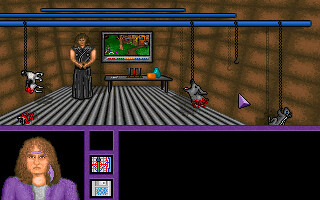In the image, to the left, there is a column of squares. The top square is black and is situated above a central square that features a navigation map. The bottom square resembles a floppy disk. A person stands to the left, adorned with a purple headband embellished with a purple feather that trails down the side. This person has brown hair falling to their shoulders, is dressed in a purple jacket over a gray shirt, and is positioned against a backdrop of brown walls. Metal poles, colored blue, extend horizontally across the top of the headband, from which various animal heads, possibly cows, hang, dripping blood onto the floor. On the right side, rats dangle from the ceiling. In the background, a gray table is visible, holding vials in red, orange, gray, and blue hues. Additionally, an image is displayed on a monitor in the background.